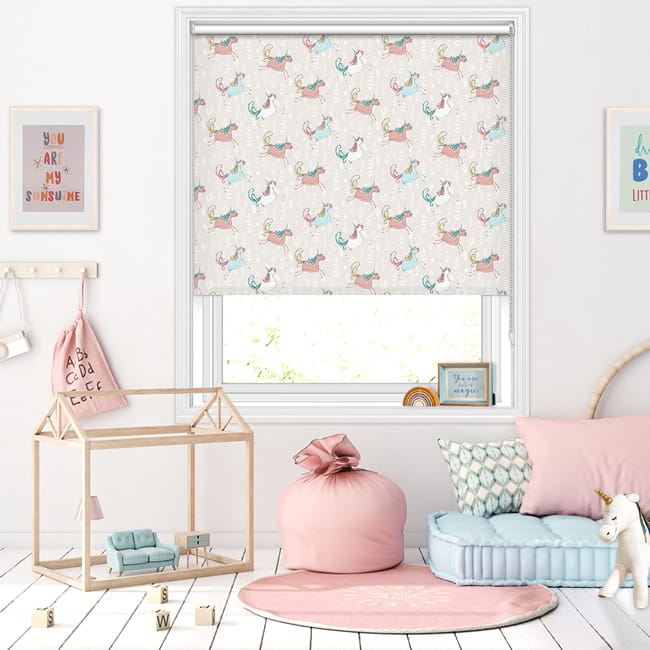The photograph captures the interior of a children’s playroom bathed in soft daylight, likely intended for a young girl. Central to the room's decor is a window adorned with pink curtains featuring whimsical animal prints and a light shade depicting pink, blue, and white unicorns, allowing a glimpse of green foliage outside. The walls are painted in a pale pink or white, harmonizing with the room's overall pink and blue theme. 

In the left corner stands a dollhouse with blue furnishings. Above it, a friendly picture frame reads "You Are My Sunshine" in multicolored letters. Below, a hanger on the wall displays a pink bag and a white toy camera. Scattered toys lie on the white wooden floor beneath a circular pink rug. Towards the right, a cozy blue bed is set on the floor, adorned with pink pillows and a white throw pillow, accompanied by a plush white unicorn. A pink bean bag adds a playful touch to the setting. Overall, the room’s decor is thoughtfully arranged to create a charming and inviting space for play and imagination.